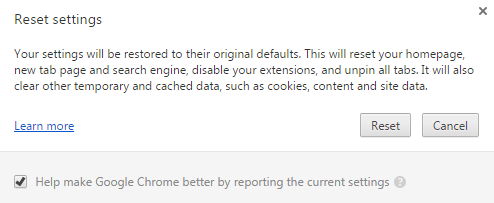Screenshot of a message regarding settings and reset options:

In the upper left-hand corner, the words "Reset Settings" appear in bold black text against a clean white background, clearly indicating the topic of the message. Below this title, detailed explanatory text outlines the impacts of resetting settings. It states: "Your settings will be restored to their original defaults. This will reset your home page, new tab page, and search engine. Disable your extensions and unpin all tabs. It will also clear other temporary or cached data such as cookies, content, and site data." 

A clickable "Learn More" link, highlighted in blue for visibility, is located at the lower left-hand corner of the text block, offering users additional information. To the right of this link, positioned side-by-side, are two buttons: a gray "Reset" button intended for executing the reset action, and a "Cancel" button for aborting the process.

Further down, a checkable grey box is included with the option: "Help make Google Chrome better by reporting the current settings," allowing users to contribute feedback to Google Chrome. The various elements are neatly organized to provide a clear and informative user experience.